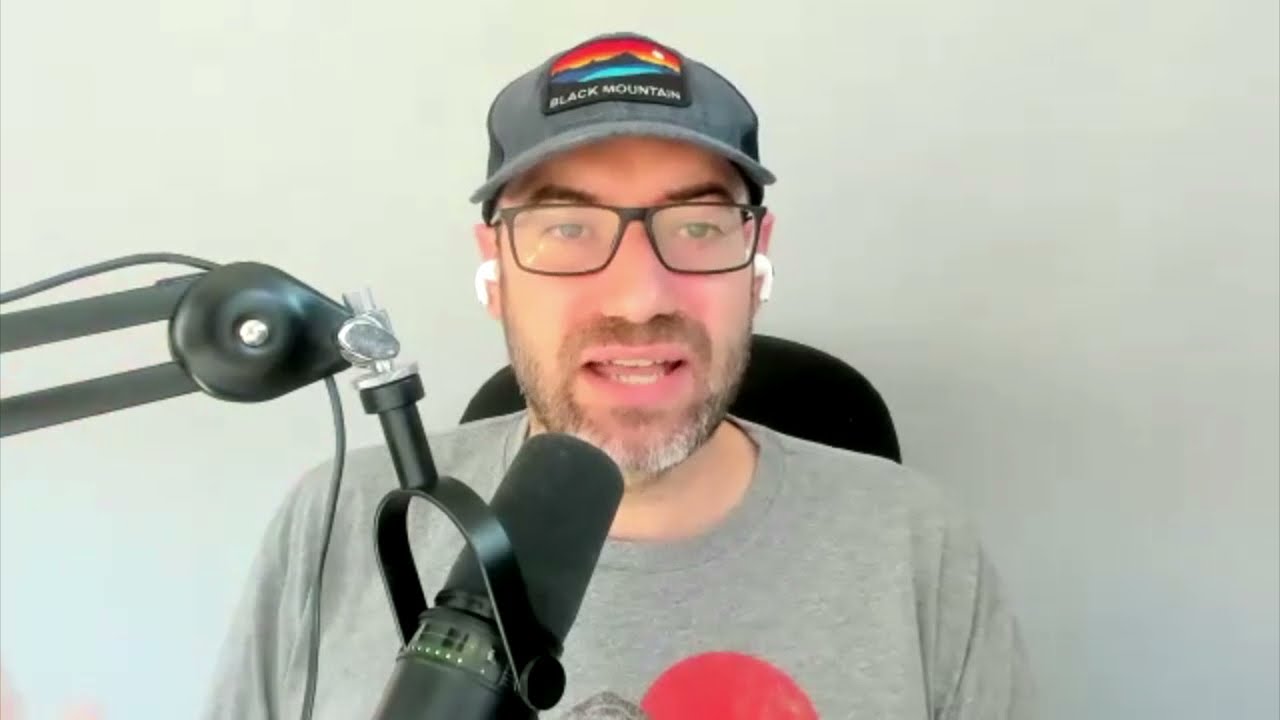The image is a still frame from a video, possibly a YouTube video or a podcast recording, featuring a white man in his early 40s. He has black-framed glasses and a scruffy beard with streaks of white predominantly on his chin, although the rest of his beard is mostly brown. He is wearing a gray t-shirt displaying a red and gray screen print on the front, and a black baseball cap with a patch that reads "Black Mountain." The patch depicts a mountain range against a red and orange sunset sky.

The man is seated in a black computer chair with a professional-grade microphone mounted on a metal arm positioned in front of him. He is wearing white wireless earbuds in both ears. The man appears to be mid-sentence, looking towards the right side of the camera, with his mouth open as if he is speaking. The background is a plain off-white or eggshell-colored wall, suggesting he is indoors.